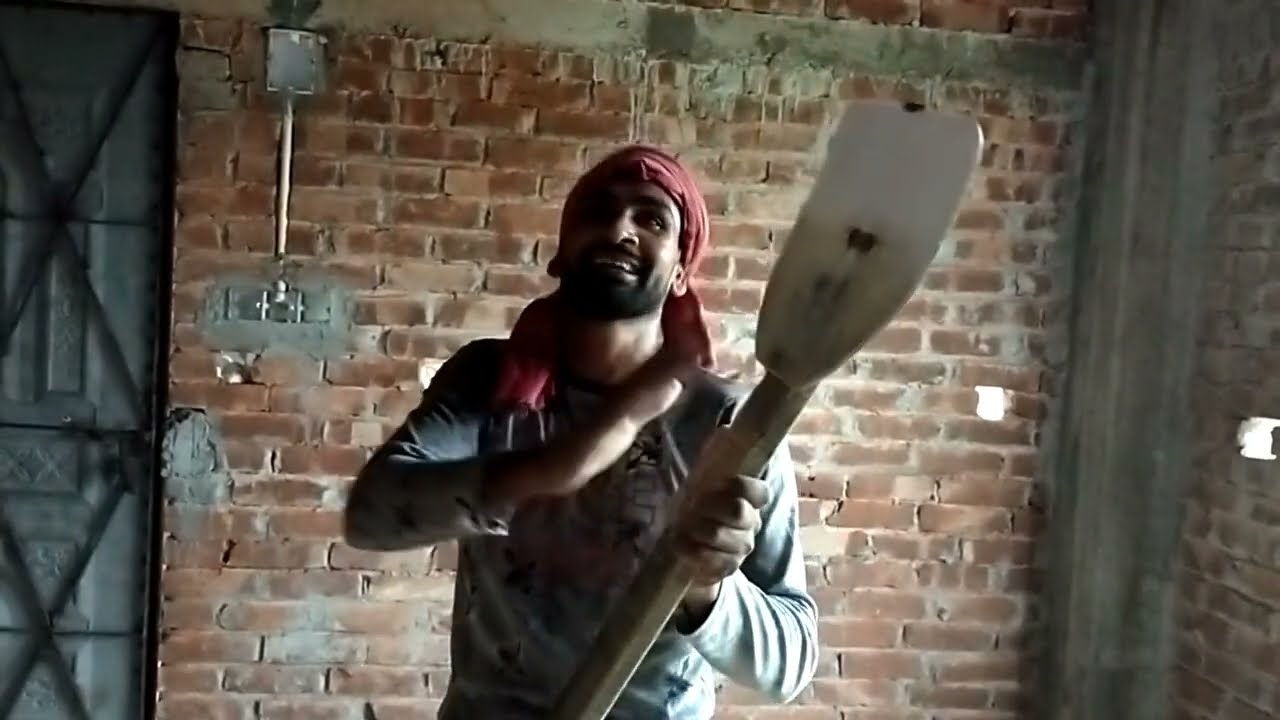In this image, we see a Middle Eastern man standing inside a dilapidated brick house with streaks of cement running down the worn-out walls. Some bricks are missing, allowing daylight to filter into the room, creating a stark contrast against the gray, decaying interior. A gray metal door frame is visible on the left side in the background, adding to the rundown ambiance of the scene.

The man is positioned centrally in the frame, smiling as he looks upward towards someone out of view behind and above the cameraman, gesturing with his right hand in mid-action. He is clad in a ribbed, raggedy, long-sleeve light-colored shirt that hints at a life of labor, and he has a distinctive dark mustache and closely shaven beard.

On his head, the man wears a red cloth, tied in a wraparound style, adding a splash of color to the otherwise muted palette of the room. In his left hand, he holds what appears to be a homemade shovel, its blade painted white and taped onto a wooden stick, though it bears a resemblance to a wooden oar. The combined elements of the man's attire, his expression, and the setting create a vivid portrayal of resilience in the face of adversity.